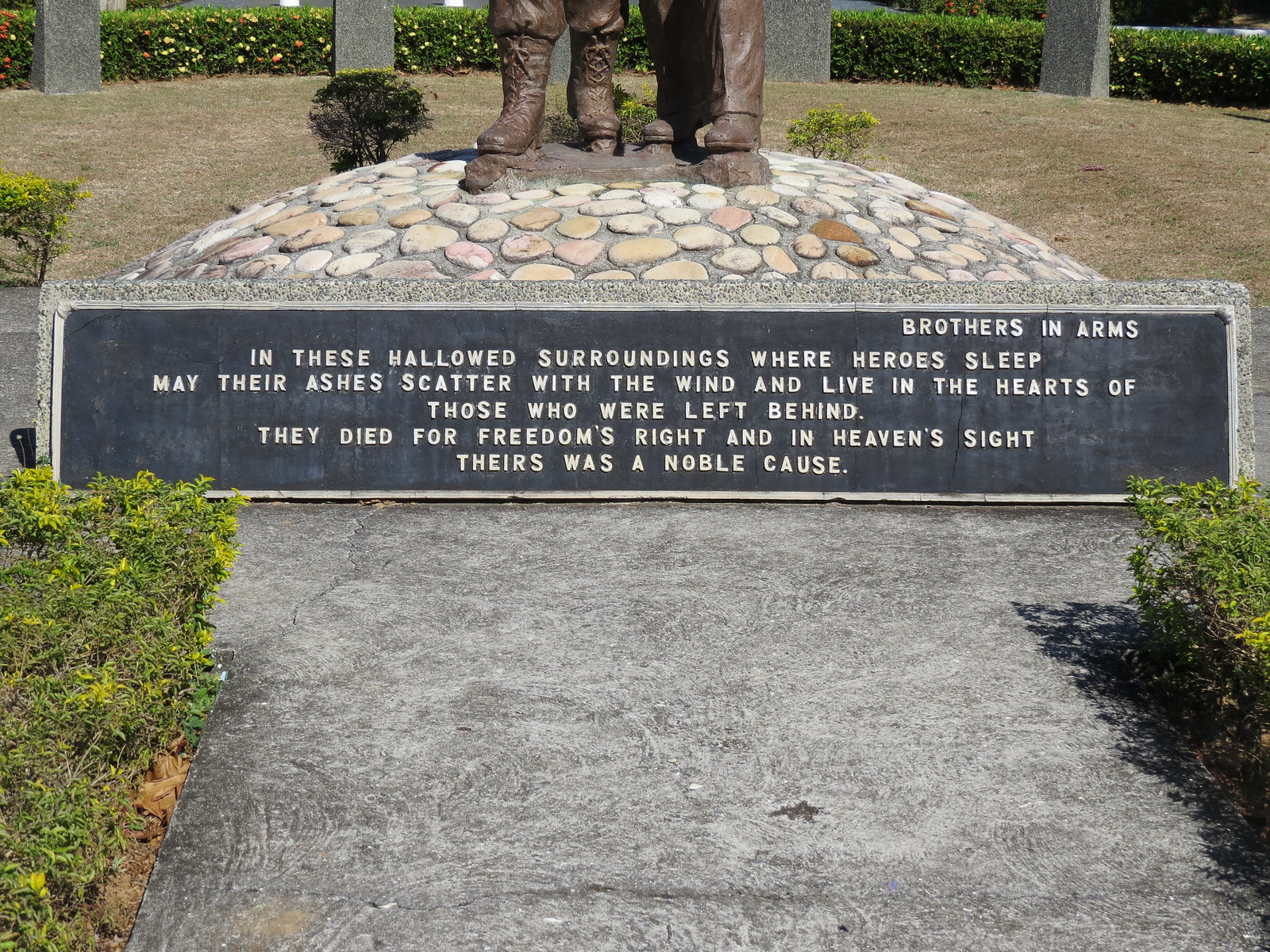The photograph depicts the lower half of a monument dedicated to soldiers, featuring their boots and feet standing on a small rocky hill. A black plaque with white raised lettering reads: "Brothers in Arms. In these hallowed surroundings where heroes sleep, may their ashes scatter with the wind and live in the hearts of those who were left behind. They died for freedom's right and in heaven's sight. Theirs was a noble cause."

The scene includes a stone or concrete path leading to the monument, flanked on both sides by patches of green grass and shrubbery. Additional bushes and green foliage are present both behind and surrounding the monument, and the photograph was taken during daylight. Other stone monuments can be seen in the background, enhancing the solemn and commemorative atmosphere of the setting.